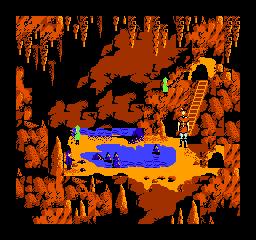This highly pixelated screen capture from a video game depicts a scene set inside a cave, featuring a predominately orange and brown color palette, highlighting the natural stalagmites and stalactites, as well as various rock formations along the edges. At the center, a male figure, lacking detailed facial and bodily features due to the resolution, stands at the base of a staircase. He is positioned on a circular, beach-like area that surrounds a blue body of water, from which more rock formations extend. Across the water, two smaller pixelated figures are visible; one is donned in a bright green coat while the other wears a blue shirt.